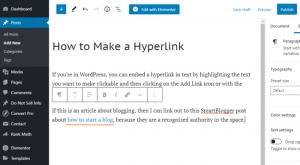This image is a heavily cropped and low-resolution screenshot taken from a webpage, resulting in a very small and blurry visual. Despite the blurriness, several key elements can be identified. On the left side, there is a menu section with a black background; although the menu items are indistinct, the top menu item clearly displays the word "Dashboard." Running across the top of the screen, there are numerous icons and a navigation menu featuring options like "Save," "Draft," "Preview," and "Publish," which are commonly associated with webpage management. The main content area prominently features a large title reading "How to Make a Hyperlink." Below the title, some text is visible, though the details are unclear. Additionally, a pop-out window with formatting options for text is present, indicating tools typically used for editing or customizing text content.